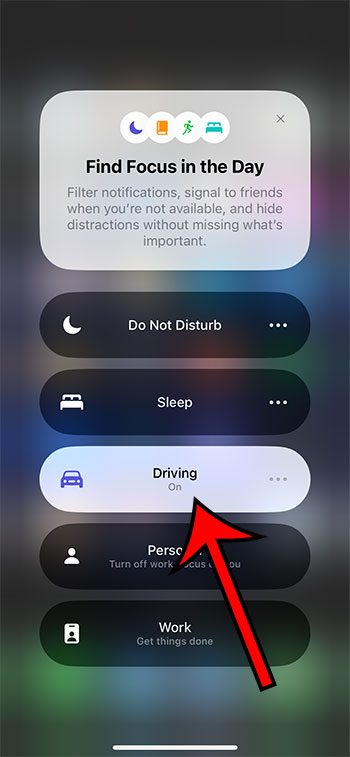This image is a screenshot of an iPhone screen displaying its various Focus modes under the Do Not Disturb settings. At the top of the screen, there is a prominent box with text providing an overview of the Focus feature. The text reads: "Find focus in the day, filter notifications, signal to friends when you're not available, and hide distractions without missing what's important."

Below this informative box, different Focus modes are listed vertically, each accompanied by unique icons and descriptions:

1. **Do Not Disturb:** Represented by a moon icon, this mode is currently not activated.
2. **Sleep:** Marked with a bed icon, indicating it is designed for sleep time.
3. **Driving:** This mode is depicted with a car icon. Notably, it is the active mode, as indicated by its white and opaque appearance, with the word "on" underneath. A large red arrow is also pointing toward this mode, emphasizing its activation.
4. **Personal:** Shown with an icon of a person and the description "Turn off work, focus on you," suggesting it is for personal time.
5. **Work:** Identified by an ID card icon, this mode's description reads "Get things done," hinting that it's for productivity and work-related tasks.

The image highlights the functionality of each Focus mode, signifying their purpose and how they can be toggled to manage different scenarios effectively. The large red arrow directing attention to the currently active Driving mode serves as a clear indicator of its status.